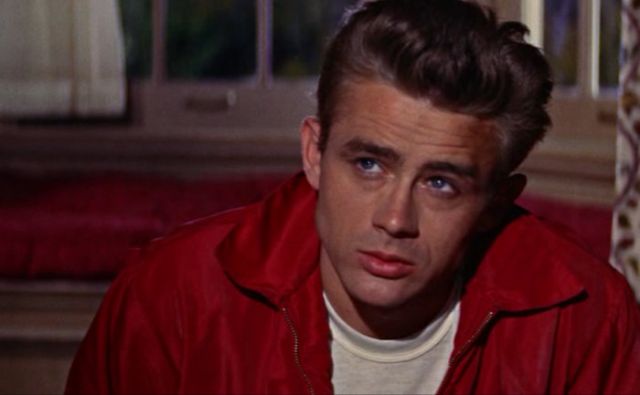The image captures a vintage scene that appears to be a still from either a TV show or movie, evoking an older vibe, possibly from the 90s or even the 50s. It features a young Caucasian man in his early 20s or 30s with dark brown hair, styled in a slight pompadour, and a few streaks of white in the front. His blue eyes, sharp nose, and pink lips are well-defined. The man is wearing a cherry red jacket, partially zipped, with a bright white t-shirt underneath. He is seated, visible from the chest up, with his gaze directed slightly upward and to the side, suggesting he's engaged in listening to someone, his expression a mix of skepticism and sadness.

The background showcases a bay window with sheer white curtains drawn to the side, allowing a glimpse of the night outside. The window frame appears brown, harmonizing with a brown podium nearby. A wine-red cushion, matching the hue of his jacket, sits at the window, adding a cozy touch to the indoor scene. The detailed setting and the man's thoughtful expression suggest a moment of contemplation within a nostalgic context.